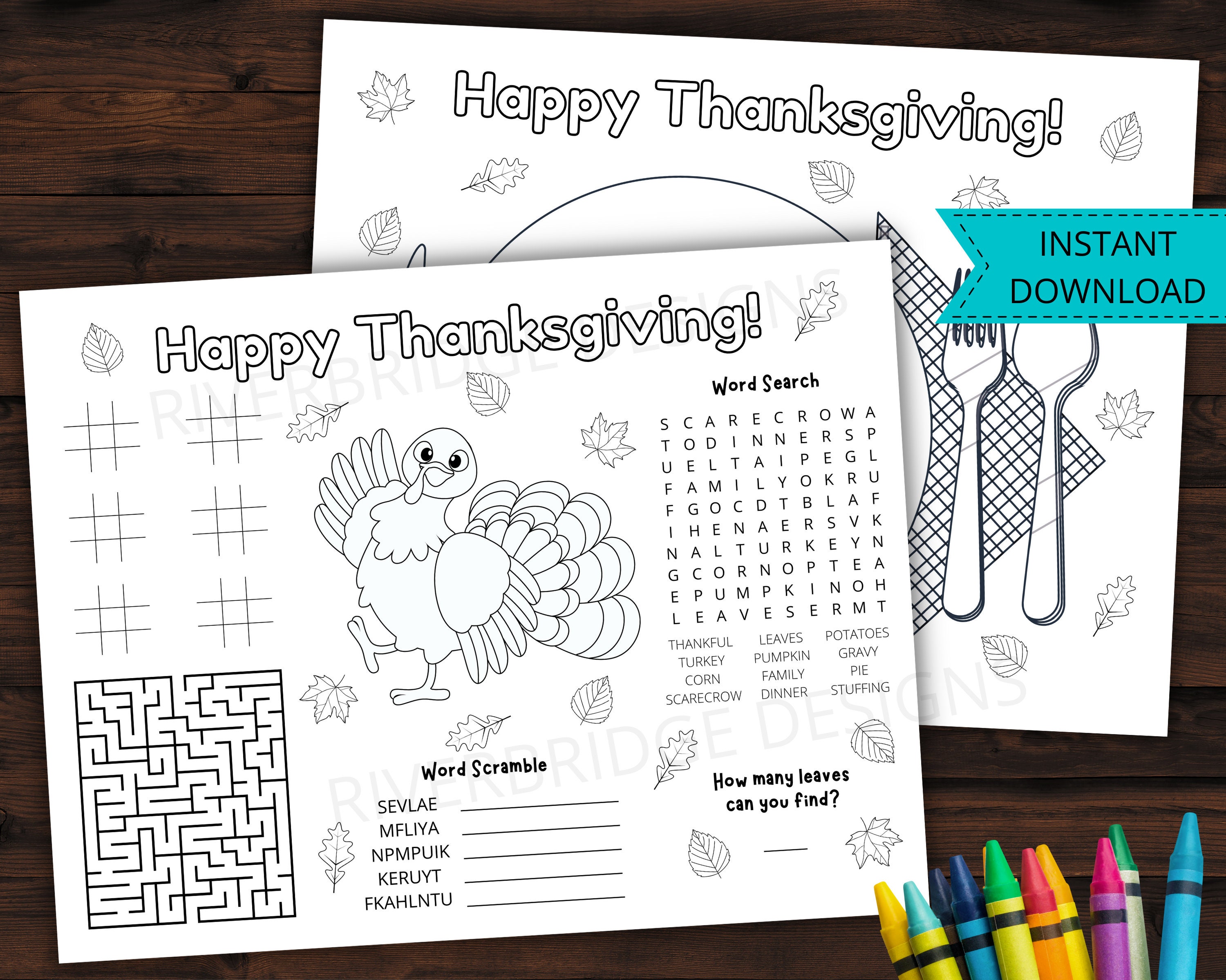The image depicts a pair of white activity sheets designed for kids, resting on a dark wooden surface with horizontal planks. The top sheet, angled slightly up from the left bottom to the right, features a variety of Thanksgiving-themed games and activities. It bears the title "Happy Thanksgiving" in bold lettering across the top. At the center is a black and white illustration of a turkey, framed by scattered fall leaves. The upper left corner contains six blank tic-tac-toe grids, while the lower left holds an unsolved maze. Below the turkey, there is a word scramble comprising five words such as S-E-V-L-A-E (leaves), M-F-L-I-Y-A (family), and N-P-M-P-U-I-K (pumpkin). The upper right corner presents a word search with twelve Thanksgiving-related words like thankful, turkey, and stuffing listed beneath it. The bottom right corner challenges kids to count the number of leaves depicted on the sheet, with a field to write their answer. Peeking from the lower right edge of the photo are the tops of some crayons, suggesting a coloring activity. The second sheet underneath, partially obscured, also reads "Happy Thanksgiving" and appears to be a placemat design with illustrations of leaves, a plate, utensils, and a black and white plaid napkin. A light teal ribbon in the top right corner of this sheet states "instant download" in capital letters.